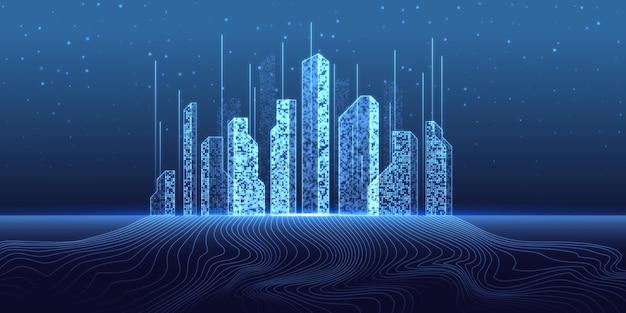The image is a digital artwork depicting a monochromatic cityscape in varying shades of blue, extending horizontally across the frame. The foreground features wavy, contoured lines that resemble either elevation maps or plant roots, possibly representing the ground. The middle of the image showcases an array of minimalist skyscrapers, each structure defined by different shades of blue and devoid of detailed features. These buildings are topped with long antennas or projections, extending vertically into the sky. In the background, the skyline is illuminated by a speckled array of stars, adding to the surreal, futuristic ambiance. The blue tonal scheme creates a cohesive, neon-like glow throughout the piece, enhancing its ethereal, night-time atmosphere.